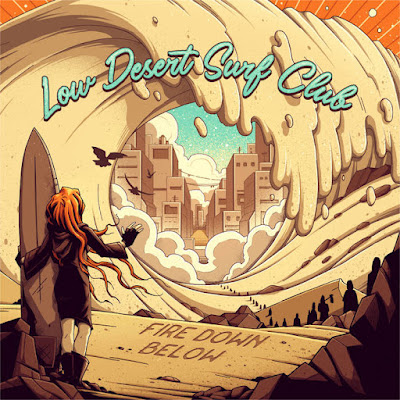The image, possibly an album cover, depicts an artistic and intriguing scene titled "Low Desert Surf Club," with the text prominently displayed at the top in a blue gradient transitioning to white. At its center stands a cartoony illustration of a woman with very long red hair, wearing a skirt or robe and knee-high black boots, holding a central-positioned surfboard. She gazes through a hole in an ocean wave that appears to be made of sand, revealing a cityscape of brown skyscrapers of varying heights within the wave. The background features an orange burst at the top left and right corners, adding a dynamic contrast. Below, on a piece of wood, the phrase "fire down below" is inscribed, hinting at an additional theme or subtitle. The image blends elements of desert and ocean, creating a surreal and evocative composition in shades of brown, with white trim and shadows adding depth.